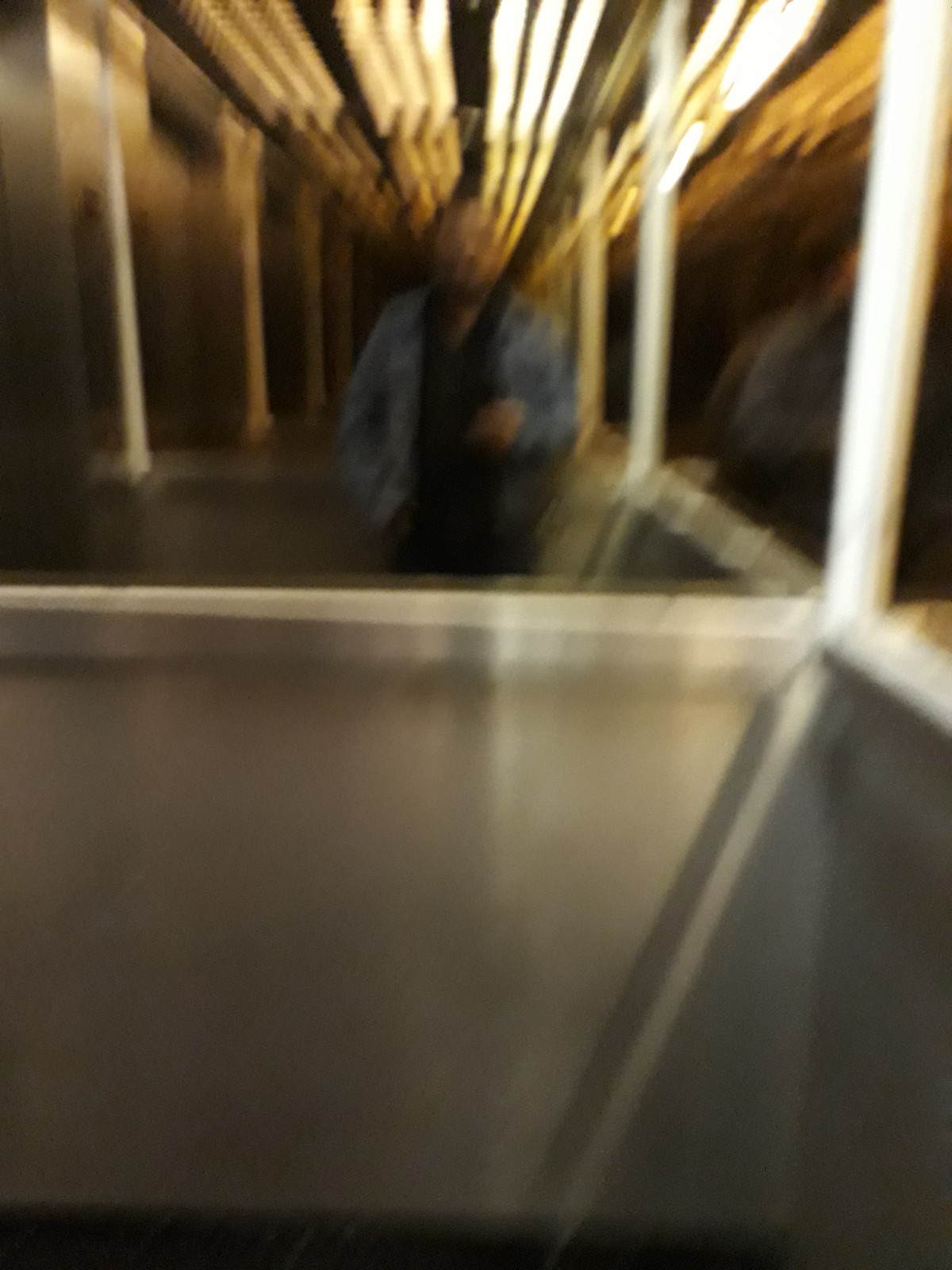In this blurred and low-quality image, a man can be seen standing in what might be an elevator or a reflective box-like area. The surroundings suggest a setting with gray, possibly metal walls and a prominent mirror. The mirror adds complexity to the scene by reflecting the man, who wears a blue denim jacket over a black shirt. His face and precise features are indiscernible due to the blurriness, but his darker skin complexion is faintly visible. His right arm is raised, with his hand appearing to rest on his chest. Above him, rows of fluorescent or round bulb lights create a repetitive, almost infinite reflection effect, amplifying the disorientation caused by the photo’s haziness. To the right, another figure seems to be present, obscured by the mirror’s reflections, giving the impression of additional booths or a corridor with windows, whiteboards, and possible posts. The man's black cell phone suggests he might be the one taking the picture, adding to the mirror's effect of repeated reflections.